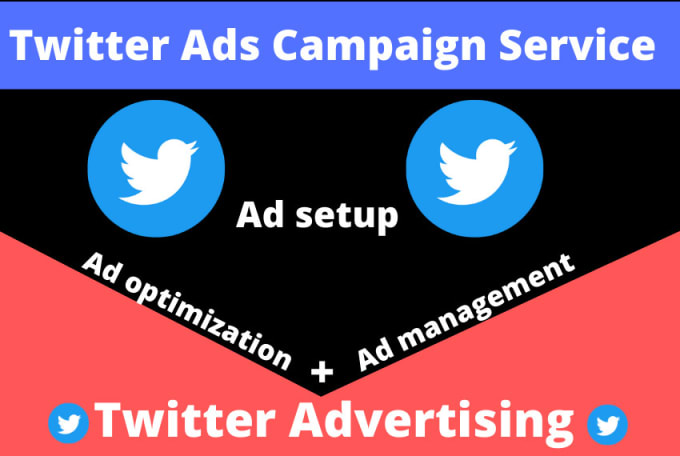### Websites

The image features a simplistic yet colorful design with a focus on Twitter advertising services. Across the top, a striking blue banner prominently displays the text "Twitter Ads Campaign Service" in crisp white letters. 

Below this blue banner, the main part of the image resembles an envelope. The flap of the envelope is rendered in black and bears the text "Ad Setup" in the middle, also in white. Flanking the "Ad Setup" text on both sides are the outdated Twitter logos, with the classic blue bird icons that have since been replaced by "X". 

Along the left edge of the black flap, the words "Ad Optimization" are inscribed, while the right edge reads "Ad Management." At the pointed tip of the flap, there's a small white symbol that reads "Plus."

The bottom portion of the envelope-like design is pink. This section also features two of the old Twitter logos in blue circles with white birds, one on each side. Along the very bottom in bold white letters is the text "Twitter Advertising."

Overall, the image is a blend of blue, white, black, and pink. The outdated Twitter bird logo appears four times, emphasizing the theme of Twitter advertising services.